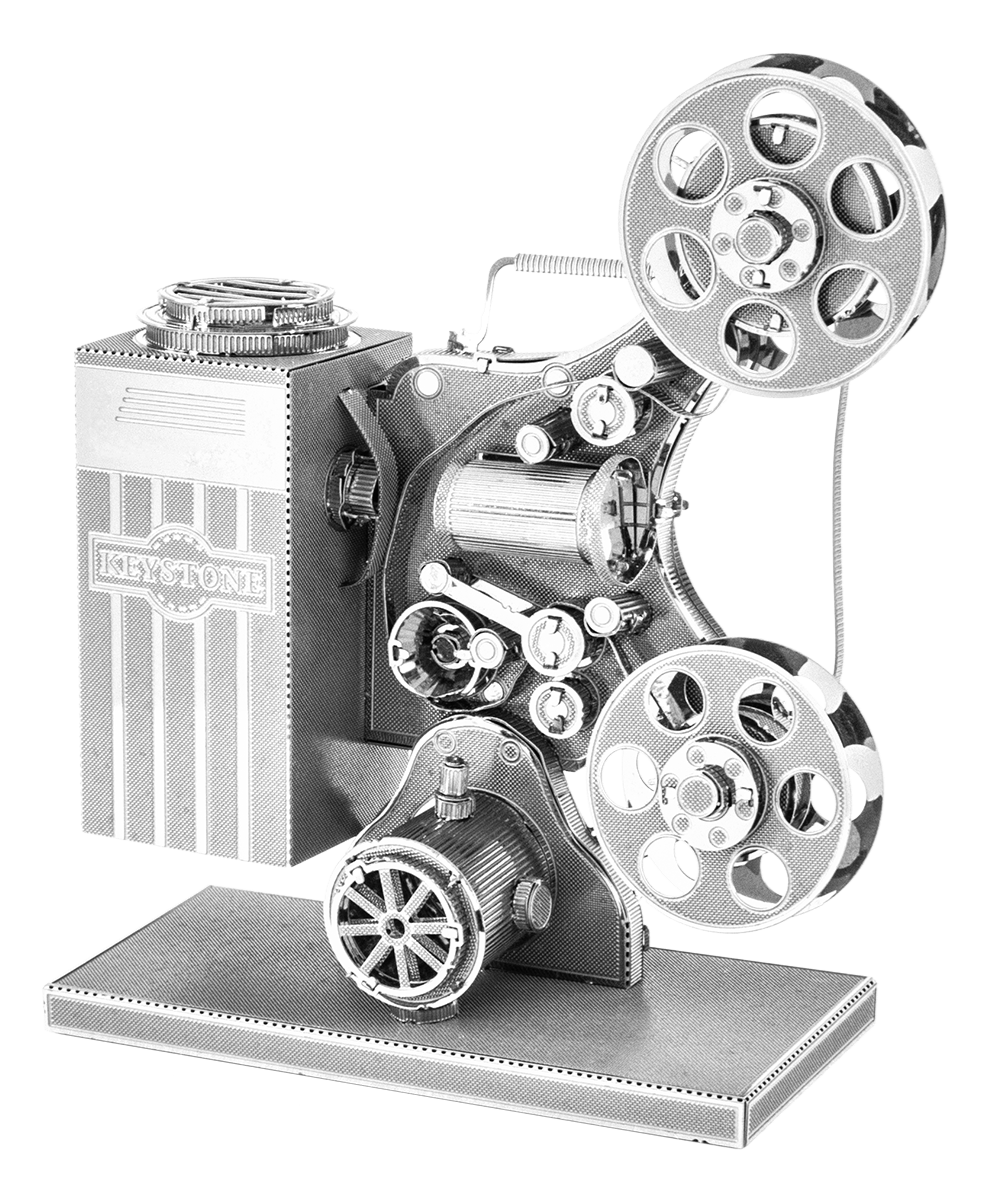The image is a highly detailed illustration, reminiscent of something you might find in a high-end magazine. It features a palette dominated by shades of silver, white, and touches of black. Central to the composition is a large, metallic rectangular structure emblazoned with the word "Keystone" and embellished with vertical stripes. Resting atop this metallic centerpiece are silver film reels, meticulously crafted to resemble the classic film reels of old.

The entire assembly rests on a sleek, silvery base that is dotted with small, black spots, adding texture and depth to the overall scene. At the forefront of the image lies the heart of this vintage setup: the projector itself. The projector exhibits an intricate cylindrical shape with glass components, from which the image would be projected onto a screen. Various knobs and dials adorn the device, evidencing its complexity and mechanical beauty. Strands of film trail from the reels, winding through the detailed mechanisms of the projector. Every aspect of the projector, from its cylinder to the multiple intricate circles, is rendered with meticulous attention to detail, making it a captivating piece for any observer.